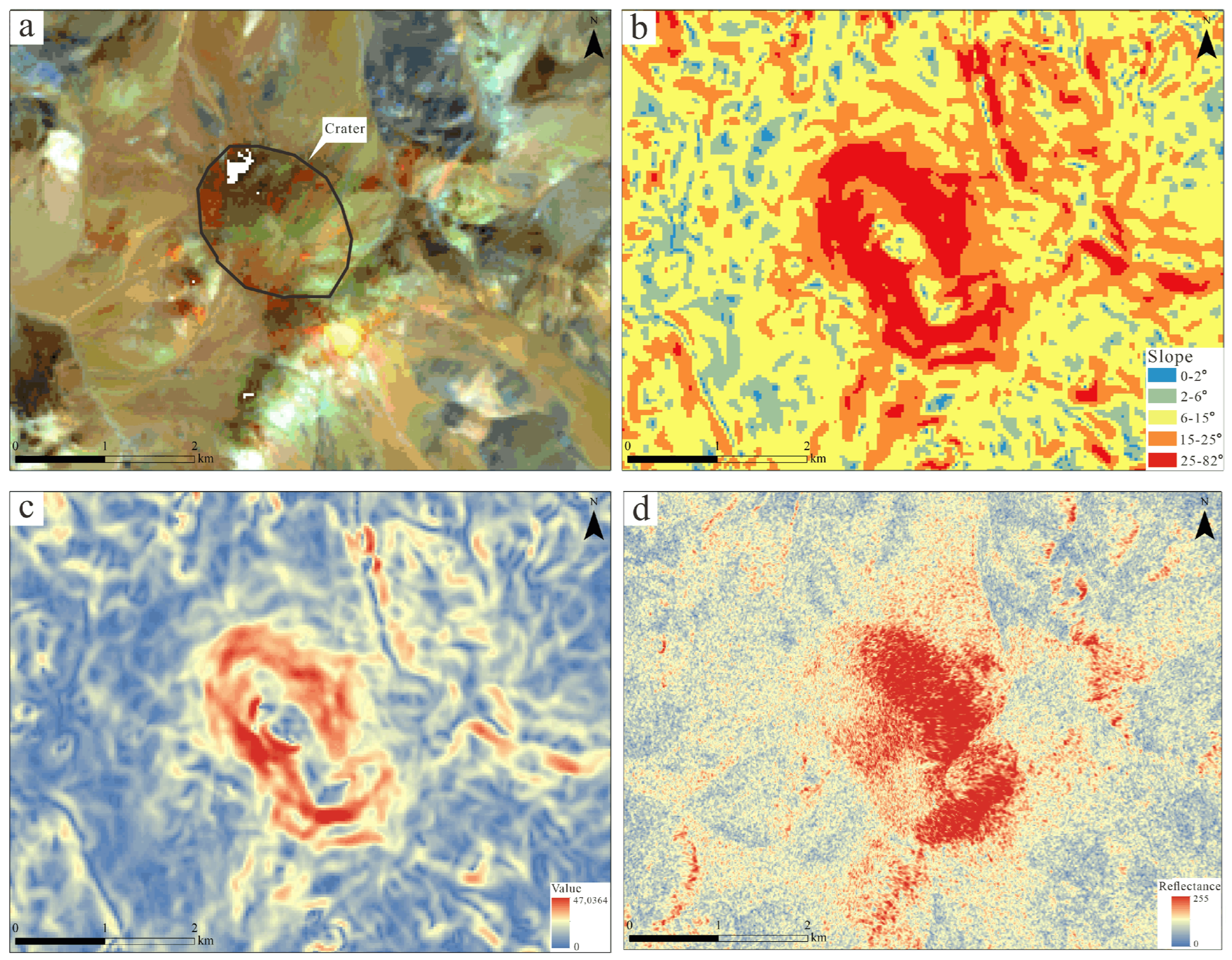This image is a detailed four-part collage, likely from Earth but possibly of another celestial body like the moon or Mars, depicting a crater site from an aerial perspective. 

- **Figure A (Top Left):** This image highlights the crater site itself, using a unique color scheme, possibly due to specialized imaging like infrared or ultraviolet. There is a scale at the bottom to provide a sense of the site's size and proportions.

- **Figure B (Top Right):** This brightly colored image represents the gradients of the slope surrounding the crater, with a key indicating the steepness of different areas. Darker colors emphasize more extreme gradients, especially near the crater, indicating steep slopes.

- **Figure C (Bottom Left):** This image maps out depth values, using a color gradient where darker colors indicate deeper sections. The crater registers as one of the deepest parts of the depicted area.

- **Figure D (Bottom Right):** This image shows reflectance values, with the crater itself exhibiting higher reflectance compared to the surrounding areas, which appear in varying shades of yellow, red, and blue.

Overall, this composite illustration effectively highlights the distinct characteristics of the crater, such as its steep slopes, significant depth, and reflective properties, setting it apart from its more gently sloping surroundings.